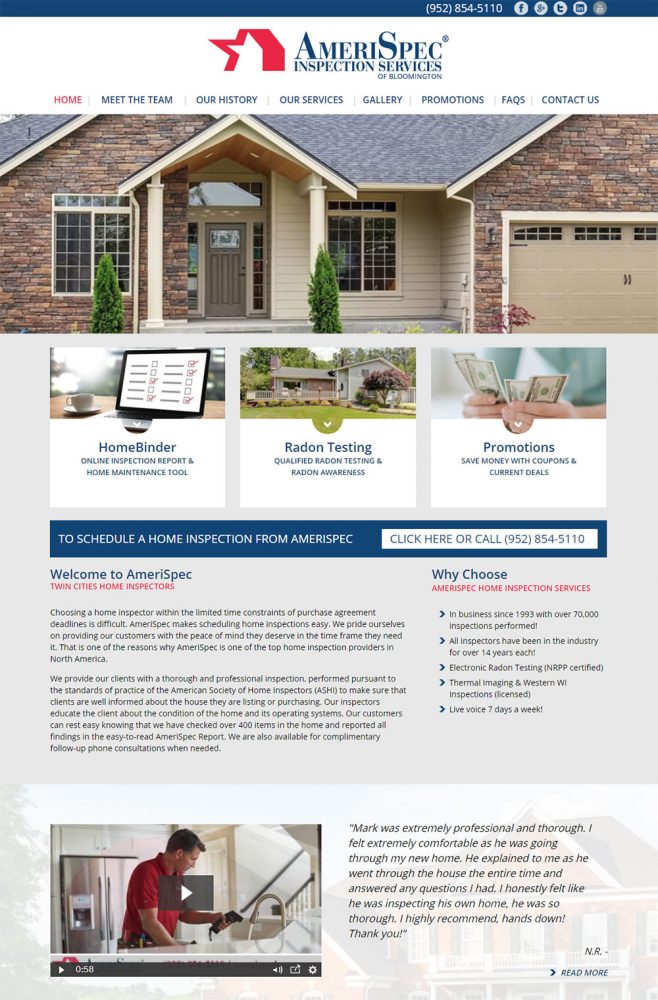The image is an online printout for AmeriSpec Inspection Services. The centerpiece of the page is AmeriSpec's red logo, prominently positioned to the left. Directly underneath the logo is a navigation bar with options such as 'Home' in red print, followed by 'Meet the Team,' 'Our History,' 'Our Services,' 'Gallery,' 'Promotions,' 'Fax,' and 'Contact Us,' all printed in a bluish hue.

Below this navigation bar, there is a featured photograph of a ranch-style home, characterized by partial brickwork and a spacious two-car garage. The house has broad windows lining the front façade, giving it a welcoming appearance.

Underneath the photograph, there's a section providing detailed descriptions and information about AmeriSpec's various services. This includes offerings such as home binders, radon testing, and ongoing promotions. An interactive section below this allows users to click for more information or to call the provided number, 952-854-5110.

At the bottom of the page, there's an area welcoming visitors to AmeriSpec, accompanied by two blurred paragraphs of text. On the left side of the lower section, there is a photo of a man standing in a kitchen. He is dressed in a red shirt and is positioned at the kitchen sink with a refrigerator in the background. This image appears to be a clickable video thumbnail, inviting users to play the video for more insights.